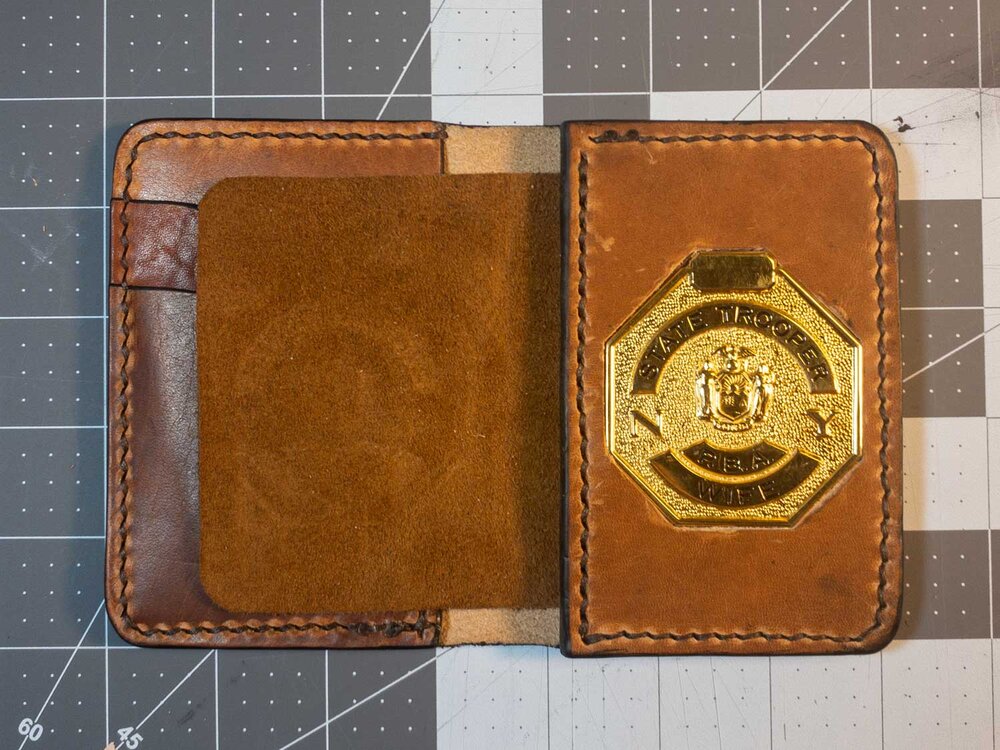The image displays a leather wallet in landscape orientation against a background of dark to light grey tiles with white dots and beige squares. The wallet, made of brown leather with dark black trim, is open to reveal its interior. The left inside flap appears to be lined with a smooth, dark brown felt, possibly suede. The right inside flap prominently features a shiny gold hexagonal badge that bears the inscription "State Trooper" along an arc, along with an insignia and additional unreadable text below. The wallet rests on a background of small, dark grey tiles that transition to light grey tiles to the right, creating a checkerboard effect.